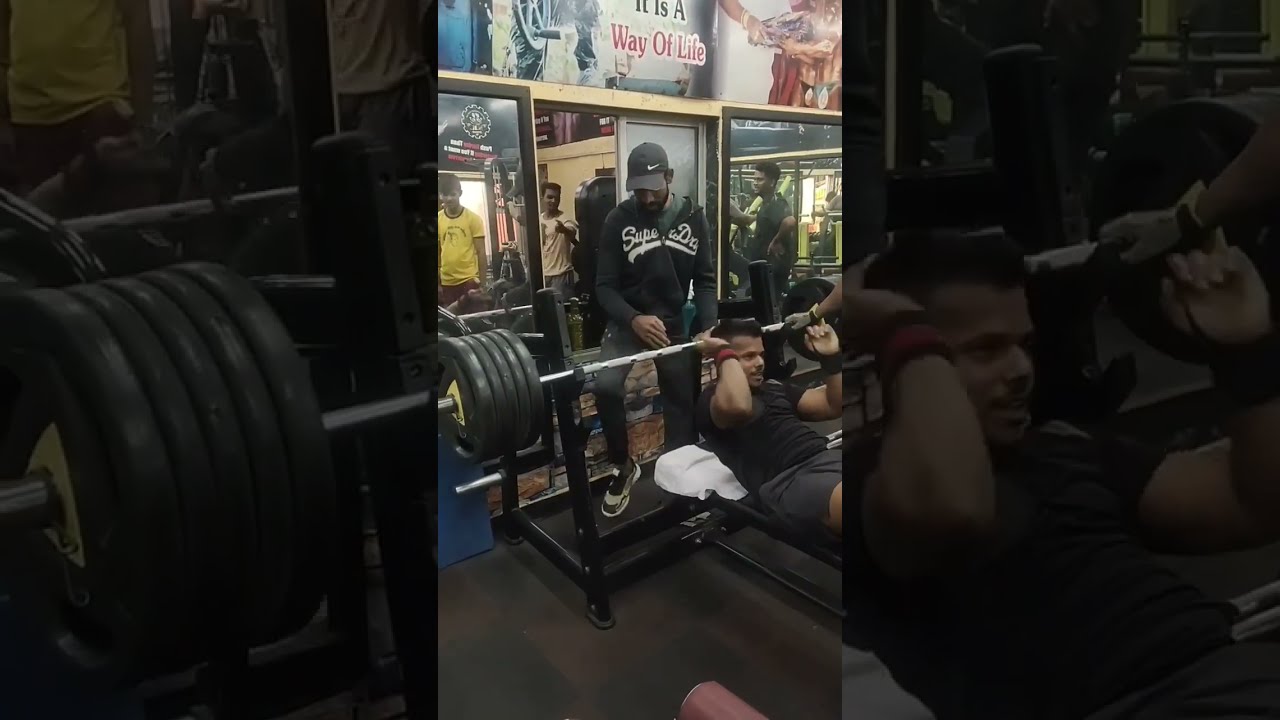The image depicts a dynamic scene in a gym, focusing on a central shot of a man preparing to bench press a significant weight. The man, with black hair and dressed in a black shirt and shorts, is captured in the moment just before he lays back on the bench, arms raised and hands positioned near his head. Behind him stands a spotter, poised and ready to assist, dressed in a distinctive Nike light gray hat and a sweater with white text.

The gym environment features large mirrors on the back wall, reflecting several other gym-goers who are observing the preparation. Above the mirrors, a prominent sign reads "It is a way of life" in bold red letters, and murals of bodybuilders embellish the upper section of the wall, adding to the gym's motivational atmosphere. A white towel is discernible on the lower right side of the central image, possibly laid across another bench or equipment.

The unique composition of the image includes a larger, underexposed version of the same scene as the background, providing a dark gray tint and a sense of depth. This layered effect emphasizes the central action and adds a dramatic contrast to the brightness of the main subject. The overall photo captures a moment full of anticipation and readiness, highlighting the culture and dedication inherent in the gym environment.